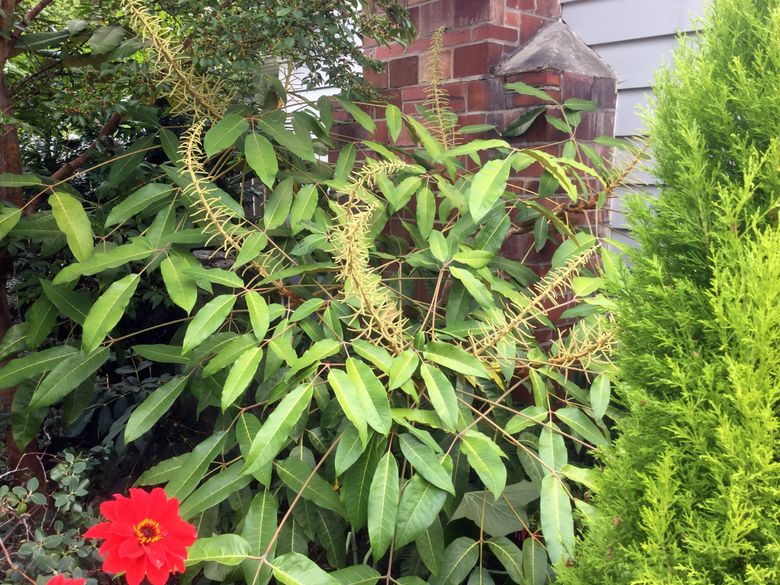The close-up photograph depicts a dense bushy area outside a house, with a mix of plants, trees, and flowers. Dominating the scene are numerous thin, long green leaves and branches with yellow protrusions scattered throughout. A bright green, young evergreen tree occupies the right side of the image, extending out of the frame at the top and bottom right corners. In the bottom left corner, a striking red flower with finger-like petals and an orangish outline stands out, partially overlapping the image's edge. Behind this vivid floral display and leafy growth, the house is visible in the background, characterized by its white wood-paneled siding and the red brick base of a chimney rising in the center. The upper portion of the image features distant treetops on the left side. The photograph is rich with textures, colors, and layers showcasing the vibrant interplay between nature and architecture.